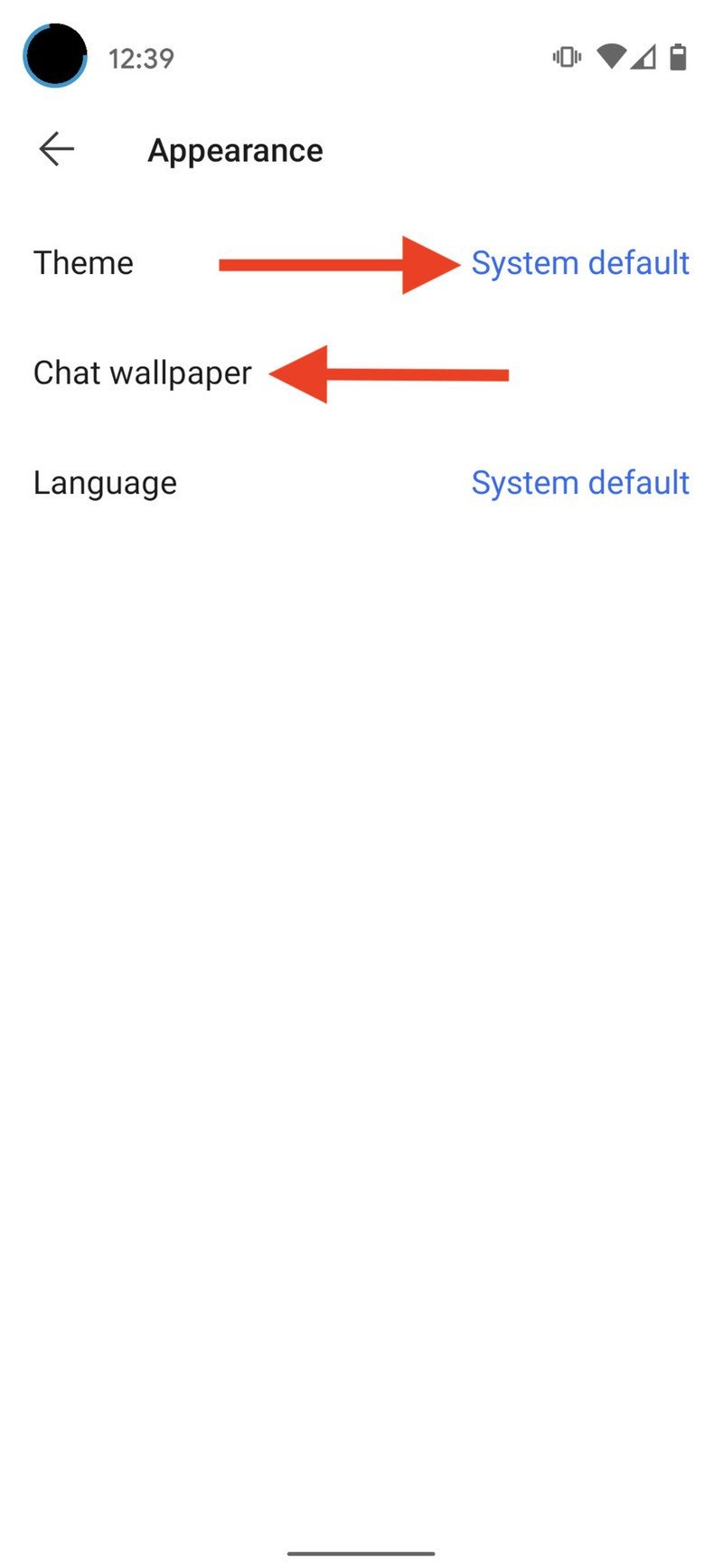This image captures a smartphone screen displaying a webpage. At the very top, the screen shows a partially enclosed black circle with a blue border, which serves as the logo. Accompanying the logo on its right are the numerals "12:39," indicating the time. Adjacent to the time display are three icons: an unknown icon, a Wi-Fi signal icon, and a battery icon displaying a half-full status.

Below the header, the screen features a settings menu. The first visible item in the menu is a left-pointing arrow accompanied by the text "Appearance," indicating a navigation option. Following this is the word "Theme," paired with a right-pointing arrow that directs to blue text reading "System default."

Further down, there is a selection labeled "Chat wallpaper," marked by a left-facing red arrow. Beneath that, another menu item labeled "Language" appears, with blue text to its right again stating "System default."

In summary, the smartphone screen presents a cleanly organized settings interface with a distinctive partially enclosed circular logo at the top, various menu options related to appearance and system preferences, and standard status icons displaying the current time, Wi-Fi connection, and battery level.